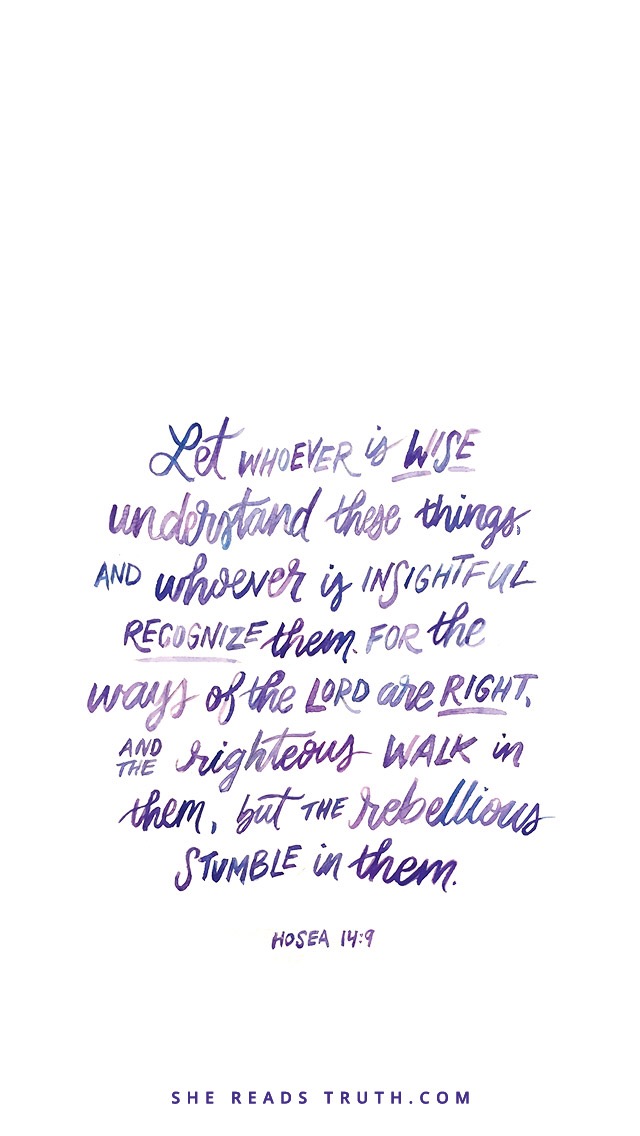The image features a white background with a visually appealing, handwritten or painted, purple watercolor text. The inspirational quote, taken from the Bible, reads, "'Let whoever is wise understand these things, and whoever is insightful recognize them. For the ways of the Lord are right, and the righteous walk in them, but the rebellious stumble in them.'" - Hosea 14:9. Below the main text, in smaller purple letters, is the URL "SheReadsTruth.com." The elegant and flowing script, which combines cursive and all-capital letters, makes the image suitable for uses such as a phone wallpaper.